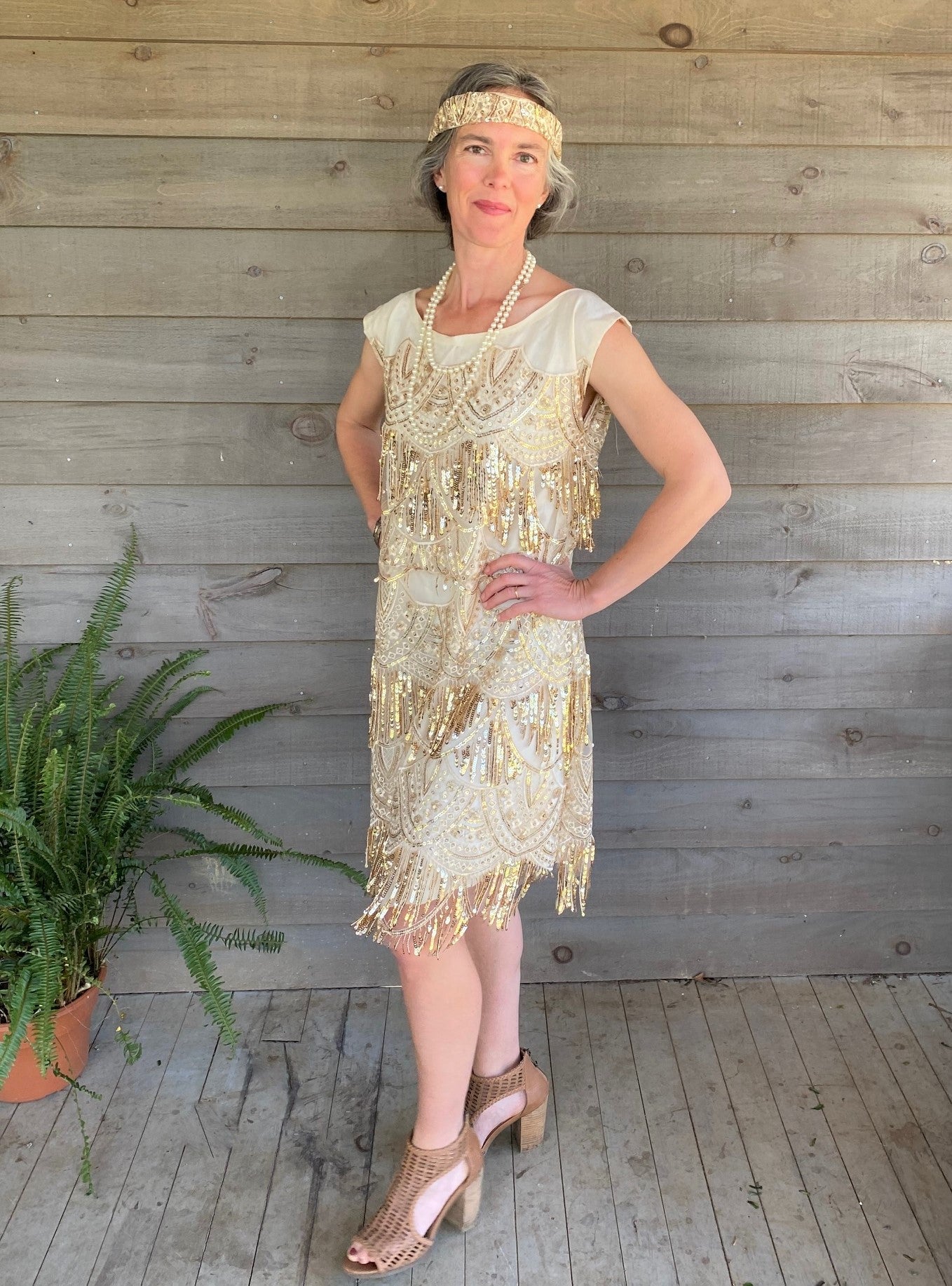The photograph captures an older woman, likely in her early 60s, with sleek gray hair styled in a short bob, elegantly pulled back. She is posing confidently with her hands on her hips and her head slightly tilted to the side. She exudes a vintage charm, wearing a stunning flapper dress reminiscent of the 1920s. The dress, which reaches her knees, is an off-white cream color adorned with intricate gold beading and sequins that cascade down, creating a delicate and shimmering effect. Complementing her dress, she wears a sequined headband that matches its aesthetic and two strings of pearls around her neck. Her footwear consists of brown, open-toed heels that blend the styles of wedges and thick heels. The setting is outdoors, featuring a backdrop of wooden planks and a wooden deck, with a potted fern placed to her left. This detailed portrayal beautifully brings out the essence of the flapper era and highlights the elegance of the woman's attire and surroundings.